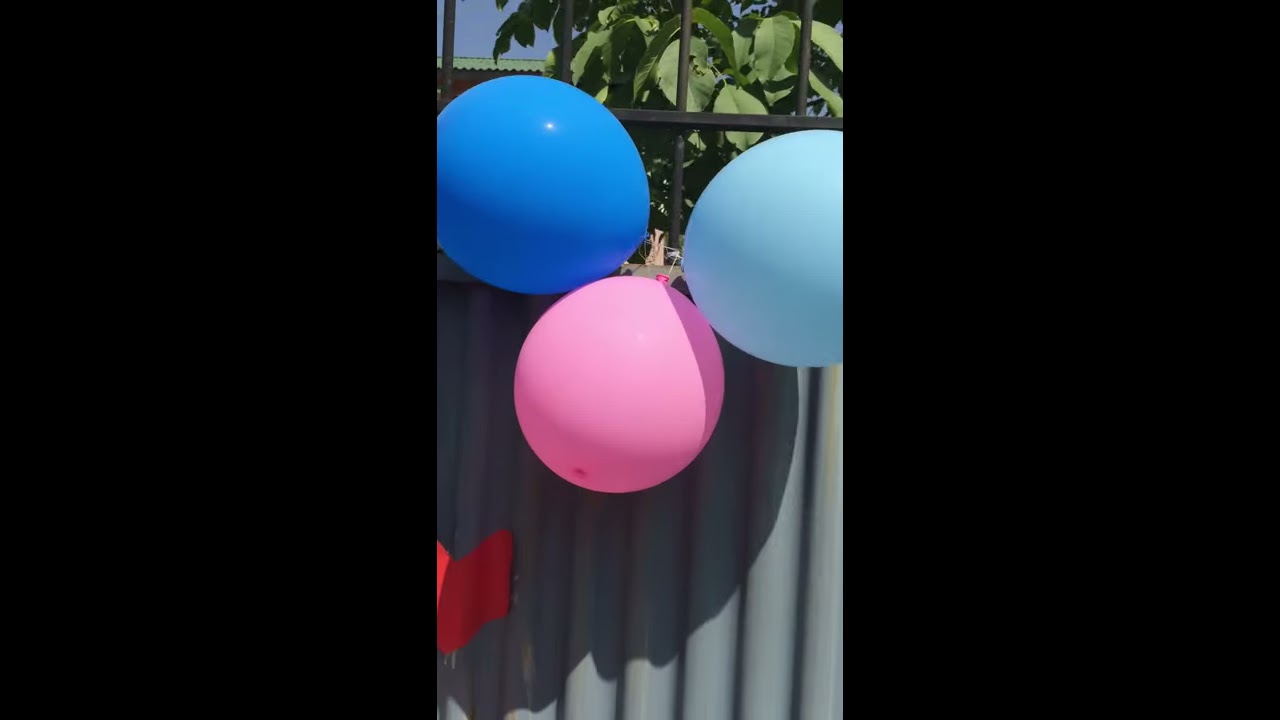The image features three balloons attached to a black metal fence with openings, allowing a view of a large leafy green plant behind it. The lower half of the fence comprises a gray corrugated metal section with a rounded texture. The balloons are arranged as follows: a cerulean or bright blue balloon on the top left, a pale pink balloon hanging downward in the middle, and a pale robin's egg or light blue balloon on the top right, which is partially cut off by the right side of the frame. Additionally, a small red V-shaped object, possibly a flag or deflated balloon, is visible in the lower left corner of the image, casting a shadow on the fence. The scene appears to be outdoors under a blue sky that is barely peeking through at the top left corner.